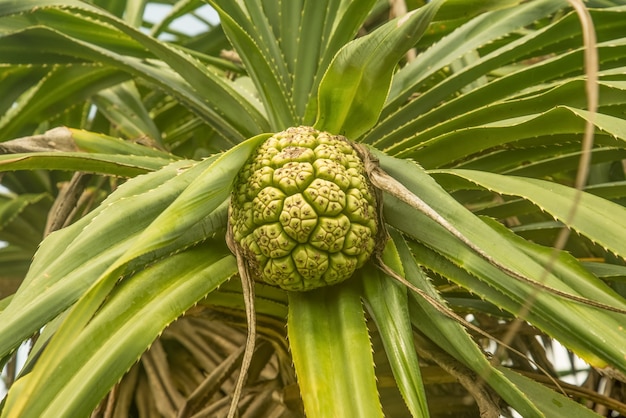The image features a strange tropical plant that evokes the appearance of aloe vera, characterized by skinny, flat-ish, and wavy leaves spreading out in all directions. These leaves are green with serrated edges, giving a rough, waxy texture. Some leaves are vibrant and green, while others appear dried and brown, indicating they are dead or dying. At the center of this plant, there is a large, bulbous fruit that resembles a mutated pineapple or a brain with its many lobes and intricate surface texture. The fruit is a yellowish-green color and significantly larger and fatter than a conventional pineapple, with sections that appear as if they could burst. The scene is set against glimpses of blue sky visible through the foliage, accentuating the exotic and somewhat alien nature of the plant.